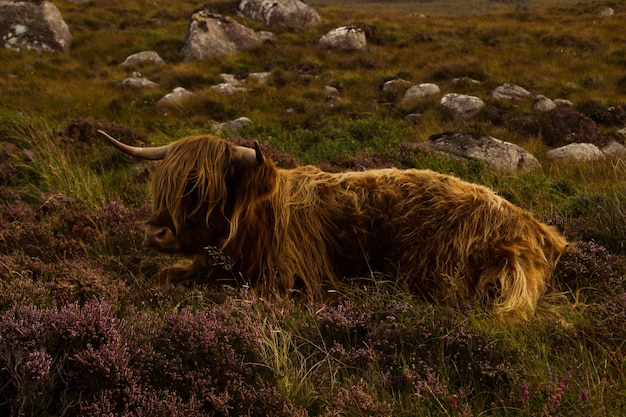The photograph showcases a Highland cattle, a specific breed from Scotland, distinguished by its long, red-brown fur that almost completely envelops its body, including the area around its eyes. This hairy bovine is likely male, discerned by its prominent, curved horns. The animal is comfortably lying down in a lush, grassy field, surrounded by a scattering of shorter green plants and delicate purple flowers. In the backdrop, several large gray rocks jut out from the landscape, contributing to the natural, rustic scene. The lighting in the image is somewhat dim, suggesting that the photo was taken either early in the morning or late in the day, casting a softer light on the cattle and enhancing the tranquil ambiance.